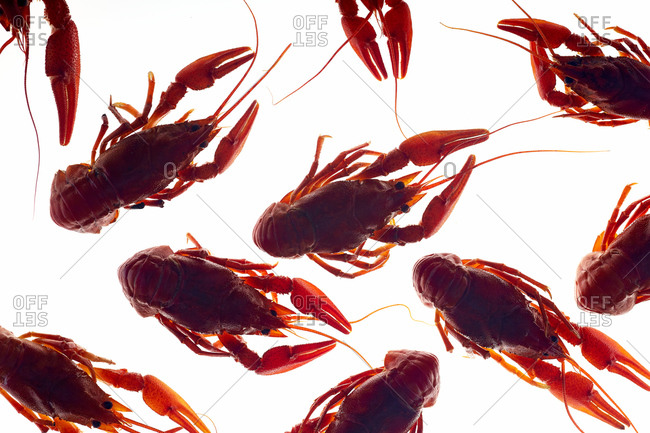The image is a stock photo on a solid white background with gray dashed lines forming diamond shapes and the word "offset" scattered throughout. It features numerous reddish-brown critters resembling small lobsters or crawdads. The creatures have elongated oval bodies with circular lines on their lower section, two long and thin front claws, beady black eyes, and antennae protruding from their mouth area. In the center of the image are four complete critters, while their partially cropped counterparts appear at the sides, top, and bottom edges of the picture. The watermark "offset" is displayed prominently across the image, enhancing its stylized appearance.